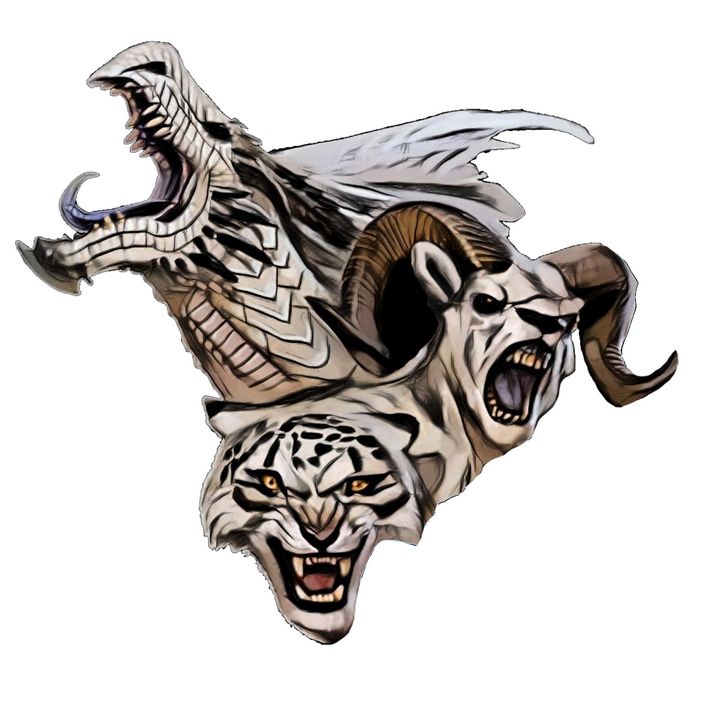The illustration appears to be a mixed-media artwork, likely executed in pen, ink, or watercolor, showcasing three fearsome animal heads set against a white background. Dominating the lower central part of the image is the forward-facing head of a leopard. The leopard's fur is depicted in a white hue with distinctive black spots, while its intense yellow eyes contrast sharply with the dark black contours around them. Its mouth is open, revealing sharp white teeth and a pink tongue.

To the right-hand side, a ram's head emerges, characterized by its prominently curled horns that spiral forward. The ram's coat is similarly in shades of white and tan, with black eyes punctuated by a tiny white speck. Its black nose and open mouth, displaying yellowish-white teeth and visible tongue, add to its fierce expression.

On the left-hand side, the side profile of a dragon's head ascends, adorned with silver scales and a distinctive, almost beak-like jaw. The dragon's mouth is wide open, showcasing numerous sharp white teeth and a long black tongue curled into a C-shape. Additionally, subtle white wings are seen extending from the back of the dragon's head. Together, these three interconnected heads form a dramatic and intense composition, unified by their shared color palette of tans, whites, and blacks.